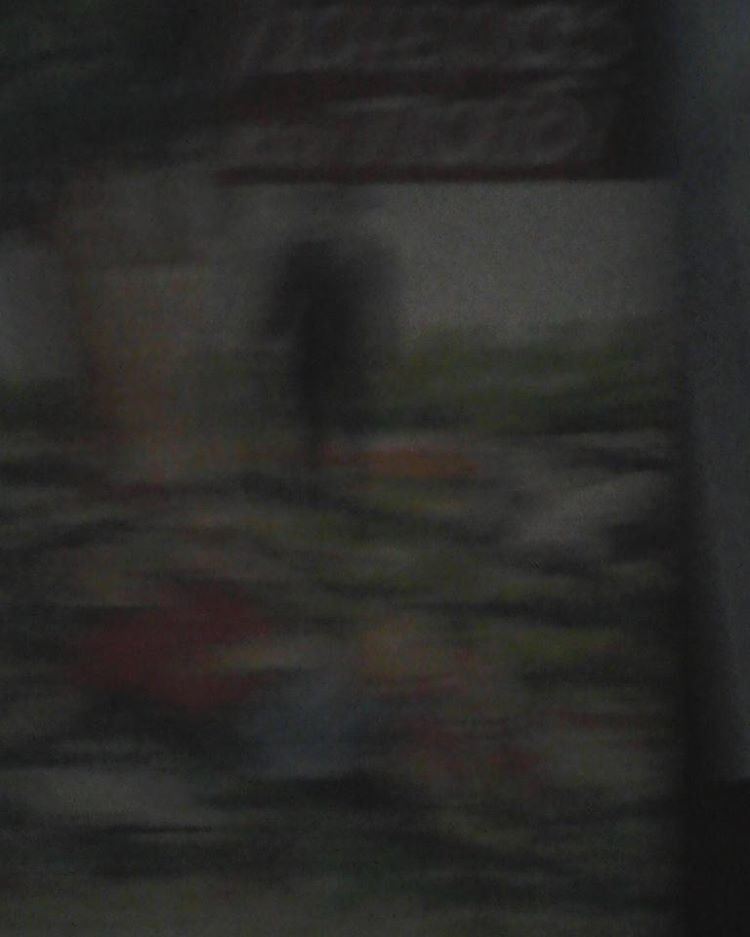This image is a very dark, blurry, and low-resolution rendition that mainly consists of indistinguishable shapes and colors. Predominantly black, it features patches and shades of blue, red, yellow, orange, and green throughout. Centered in the vertical, portrait-oriented frame is a black shape that suggests a silhouette of a person, possibly wearing a black suit or clothing. The figure might be standing over or near what could be interpreted as green scenery. Surrounding the indistinct central figure, there are occasional squiggly horizontal lines, areas that might be lighter at the top—perhaps the sky—and scattered color highlights including white, green, and red. Overall, the image remains highly abstract and ambiguous, making precise details difficult to discern.